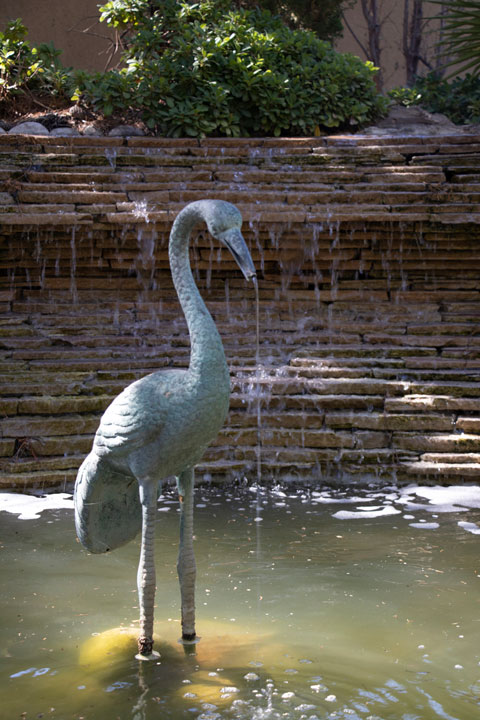A color photograph captures a serene fountain scene featuring a striking statue of a bird, likely a crane, egret, or heron, standing in a shallow, murky, greenish-brown pond. The bird, which has a long neck and legs and is made of a cream or verdigris-covered material, appears somewhat greenish-gray, possibly due to weathering. Water flows gently from its beak, trickling back into the pond below. The fountain is carefully crafted with layers of white and brown stones, designed so that water cascades down these bricks rather than spraying upward. Surrounding the fountain is lush vegetation, including several large, full trees and various plants atop a tall stone or log wall, suggesting this pond is part of a recessed pool, potentially viewable from an upper level walkway. The overall atmosphere suggests it is either spring or summer, adding to the tranquil, naturalistic setting devoid of people or visible signs. At the base of the bird's legs sits a green object, possibly a ball or bobble, adding a touch of intrigue to the scene.